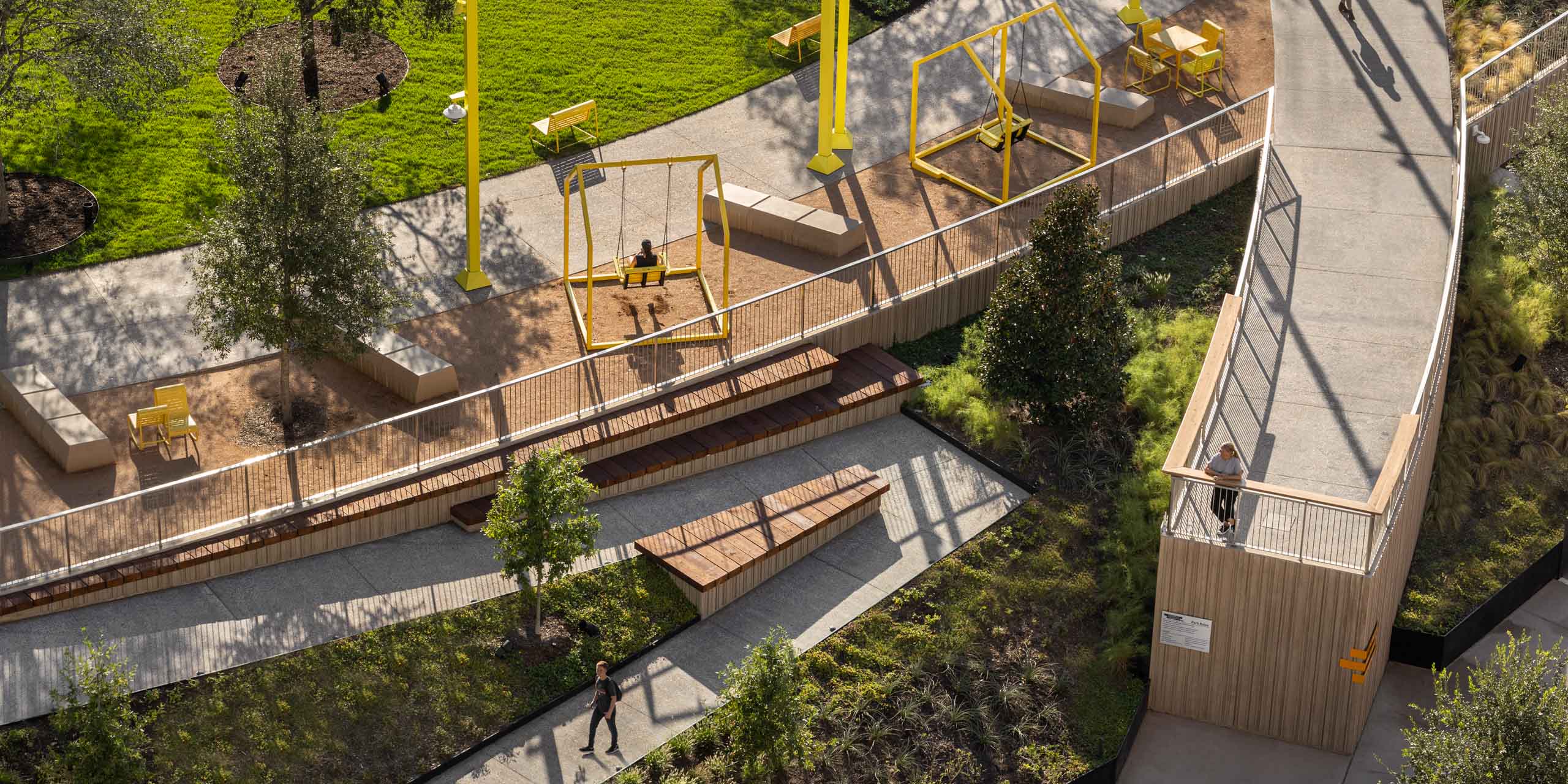The image depicts a vibrant park scene with a mix of lush green spaces, wooden sections, and concrete sidewalks. In the foreground, there is a distinctive crisscrossing walkway, where a single person is seen walking near the bottom left. Adjacent to the walkway, a white fence extends across the photo, enhancing the park's orderly layout. Beyond the fence, playground equipment is visible. Central to this area is a yellow swing, occupied by a person facing away from the camera, with an empty yellow swing to its right.

In the upper portion of the image, another paved path extends in front of the swings, leading to a green meadow that features scattered yellow benches. No people are sitting on the benches. On the right side of the image, a small outcropping of the sidewalk meets a railing, where a person is leaning, gazing over the park. The park is further characterized by smaller trees dotted throughout, and the bright green meadow is bordered at the top left by a curved sidewalk. The scene is lively yet tranquil, with three people in various activities, accentuated by vibrant yellow playground elements and the natural greenery surrounding them.